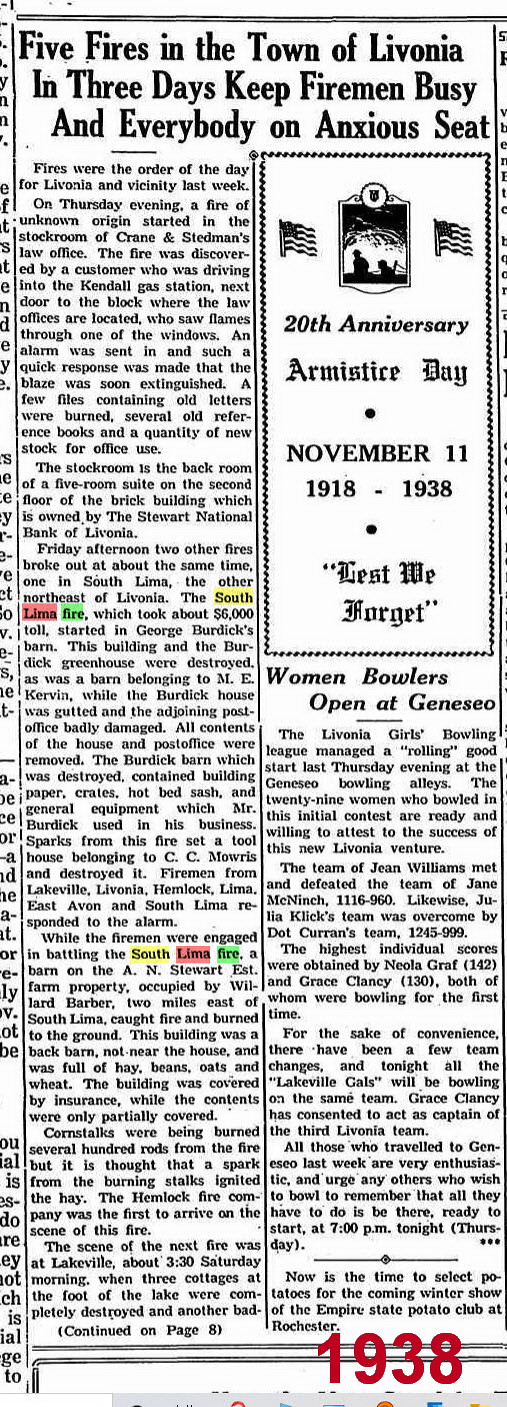The image shows a vintage, black-and-white cutout from a newspaper with a portrait orientation, spanning two columns. Dominating the top in bold black letters, the headline reads, "Five Fires in the Town of Livonia in Three Days Keep Firemen Busy and Everybody on Anxious Seat," with parts of the text highlighted in yellow, pink, and green markers. Below the headline, the left column consists of roughly five paragraphs of detailed article text. 

On the right, at the top, there is a box outlined by text, featuring an illustration of soldiers flanked by two small American flags. The text within the box commemorates the "20th Anniversary, Armistice Day, November 11, 1918 to 1938," followed by "Lest We Forget." Below this, another headline reads, "Women Bowlers Open at Geneseo." The article concludes at the bottom with a red date stamp, marked "1938."